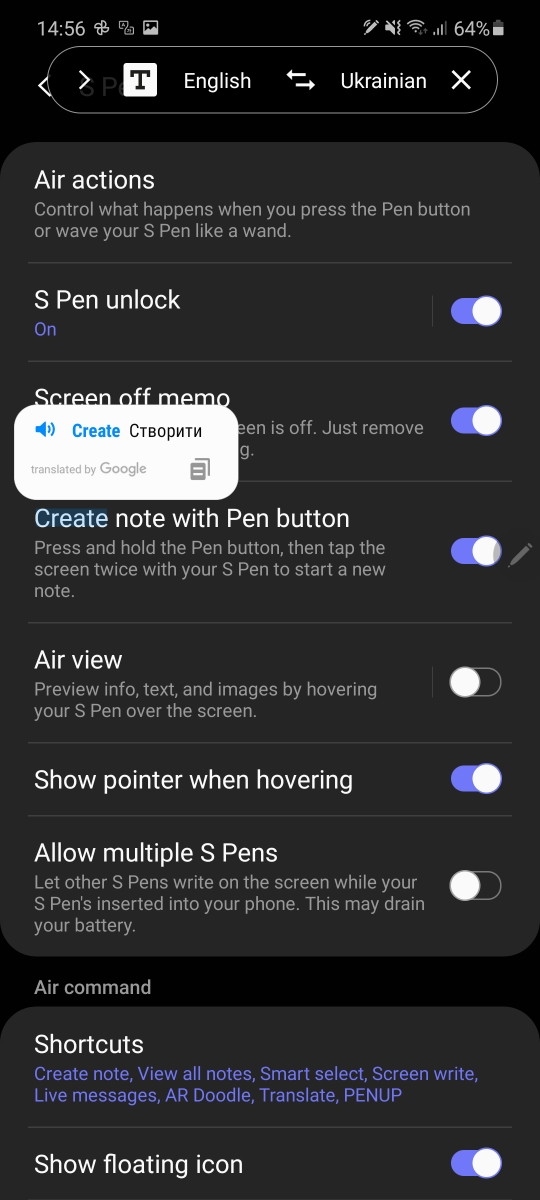A screenshot taken from a smartphone displays the language and keyboard settings in dark mode, featuring a black background with white text. The top bar contains typical phone icons: the time (14:56), a 64% battery indicator, and miscellaneous system icons. Below this, a title bar features a text icon showing a white square with an uppercase "T" and the word "English" next to it. To the right, an arrow icon indicates language translation options between English and Ukrainian.

Beneath the title bar, a series of settings pertain to the S-pen functionalities. The first setting, "Air actions," allows control over the phone using the S-pen button or gestures and is followed by "S-pen unlock," which is enabled. The "Screen off memo" setting is partially covered by a translating tool interface. This interface includes a white rectangular box with rounded edges, containing a speaker icon, the word "create" in blue bold text, and a Cyrillic word, likely Ukrainian, marked "translated by Google."

Further settings include:
- "Create note with pen button" (enabled): Allows note creation by pressing the pen button and tapping the screen twice.
- "Air view" (disabled): Previews info, text, and images by hovering the S-pen over the screen.
- "Show pointer when hovering" (enabled): Displays a pointer when the S-pen hovers above the screen.
- "Allow multiple S-pens" (disabled): Permits other S-pens to write on the screen when the primary S-pen is inserted, potentially draining the battery.

At the bottom, the "Shortcuts" section lists various quick actions including "Create note," "View all notes," "Smart select," "Screen write," "Live messages," "AR Doodle," "Translate," "Pen up," and the enabled "Show floating icon" feature. All these options are aimed at optimizing the S-pen's usability on this device, potentially a Samsung Galaxy phone or tablet.